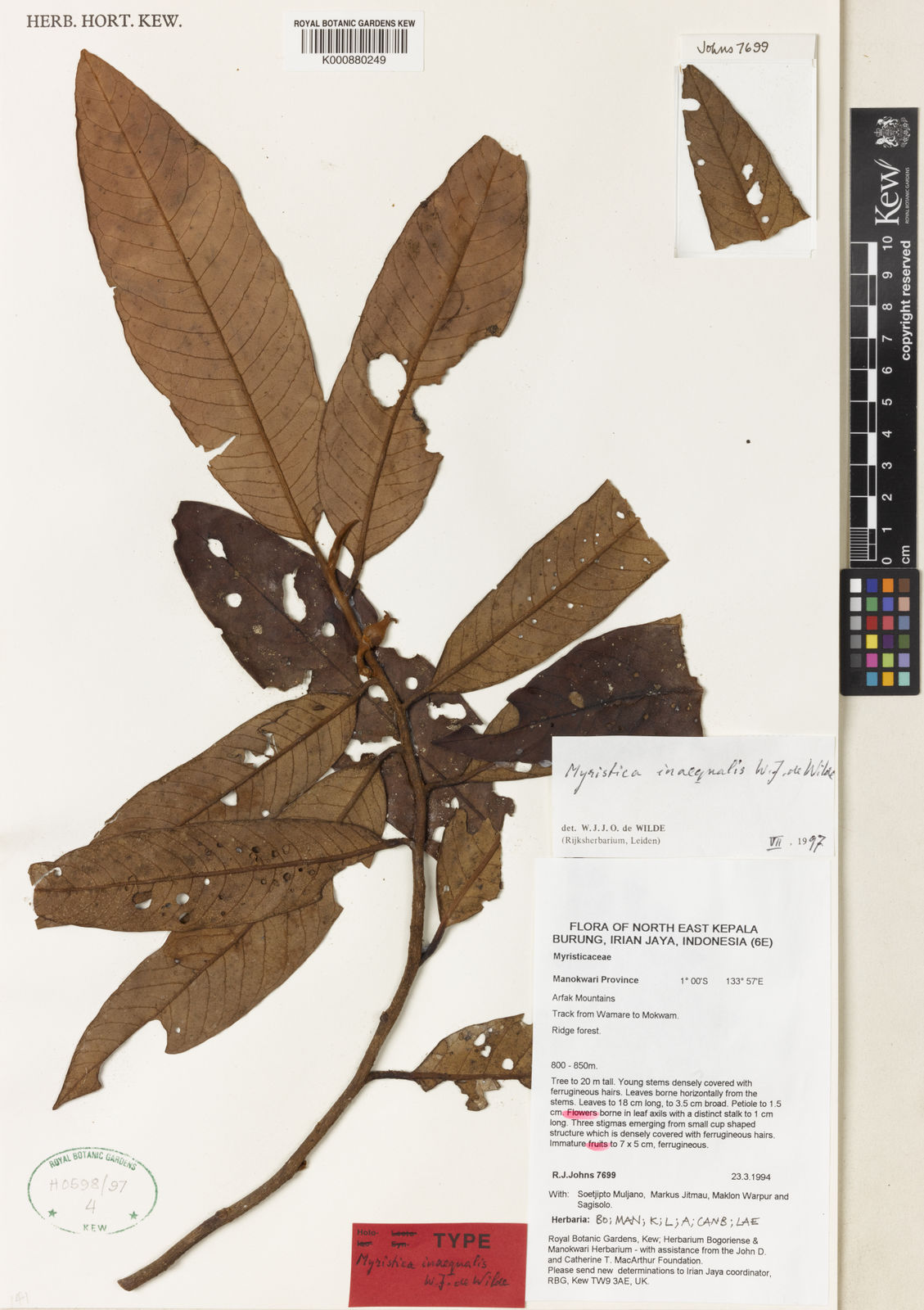This is an image of a botanical specimen from a horticultural journal or botanical brochure. The photograph is in portrait orientation and captures a yellowed piece of paper against a white background, featuring a dried branch of a plant. The branch occupies the majority of the photo and bears numerous elongated, oblong leaves that range in shades from dark chocolate brown to lighter tobacco brown, indicating they are all dead. Some leaves are severely flattened and show signs of pest damage, with visible holes and eaten-away portions. 

A black ruler and a color guide are positioned on the right for size and color comparison of the specimen. In the upper right corner, a separate piece of a leaf is enclosed in a block. The leaves display a prominent central vein with subsidiary veins extending at diagonal angles. Text on the page identifies this specimen as originating from Northeast Kapala, Indonesia, and further describes the leaf and plant characteristics. Additional notes include a red sticker at the bottom center labeled "type," along with handwritten details. In the top left corner, it mentions "herb court Q," indicating it is a referenced specimen in the Kew Gardens collection.